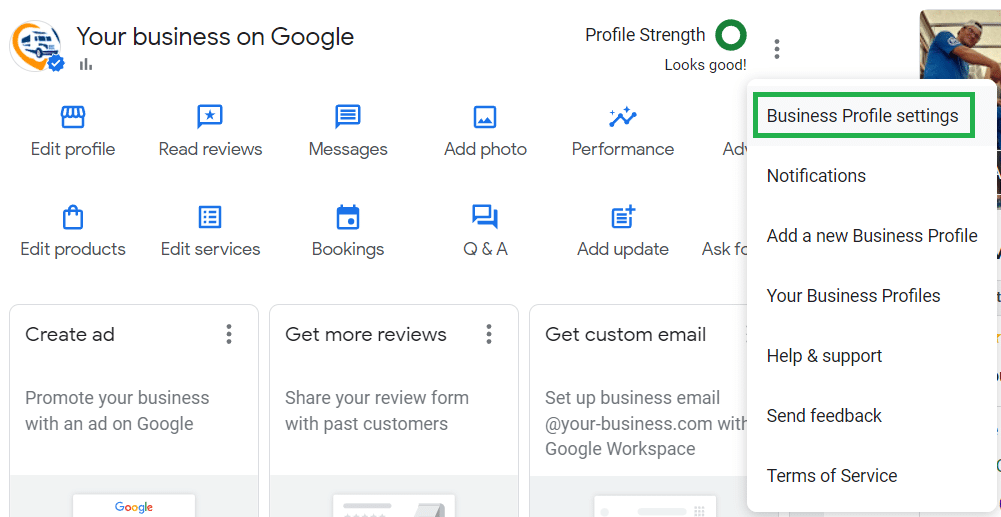This detailed screenshot captures the Google Business Profile interface on a user's desktop. In the top left corner, under the "Your business on Google" heading, the interface indicates a strong profile with a green circle and a white space in the middle. Below that, it reads "Looks good." To the right, there are three vertical dots (a menu icon), followed by a user profile picture of a man wearing a blue shirt and a white baseball cap turned backward, with the visor resting on the back of his neck.

Adjacent to the "Your business on Google" section, several options are clearly visible: "Edit profile," "Read reviews," "Messages," "Add photo," "Performance," "Edit products," "Edit services," "Bookings," "Q&A," and "Add update." To the right, a vertically positioned rectangular selector highlights the currently chosen option.

In this case, "Business profile settings" is selected, enclosed in a green rectangle with a white background. Below this section, options such as "Notifications," "Add a new business profile," "Your business profiles," "Help and support," "Send feedback," and "Terms of service" are listed. 

On the left foreground, additional options for managing and promoting the business are present: "Create ad" to promote the business using Google Ads, "Get more reviews" to share a review form with past customers, and "Get custom email" to set up a business email via Google Workspace. 

This screenshot provides a comprehensive view of the features and settings available to manage and enhance a Google Business Profile.